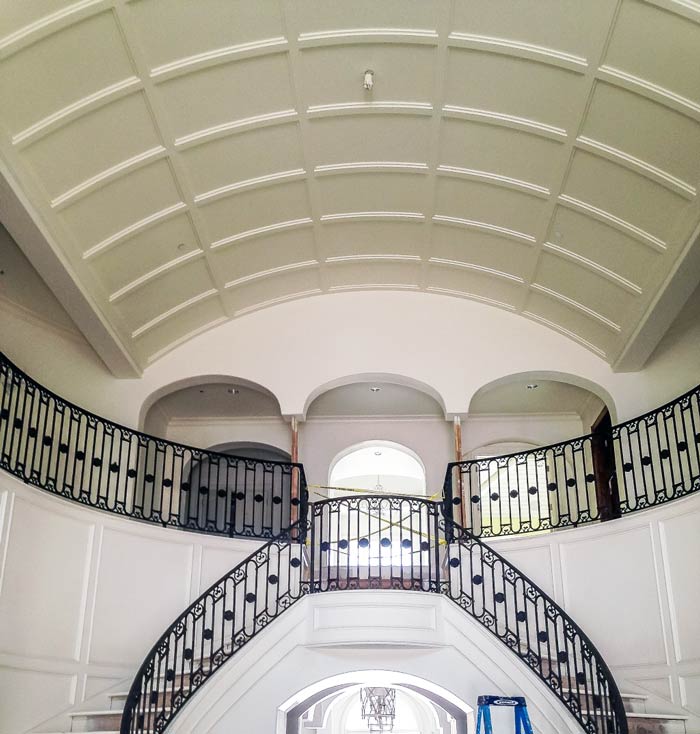This image captures the opulent interior of a large, ornate main hall in a home. The room features soaring, curved ceilings adorned with intricate crown molding. Central to the space are two elegantly curved staircases with black, ornate railings that ascend to a second-floor foyer, where the railings extend along the upper level. The second floor showcases three arched doorways: one leads to a brightly lit room, another has a closed door, and the third offers a wide-open entryway. The bottom of the image reveals a bright arched doorway leading to a room with a chandelier, as well as the visible top of a blue ladder. The ceiling's detailed woodwork adds to the room's grandeur. The house appears to be either under construction or undergoing renovation, as suggested by its partially unfinished state.